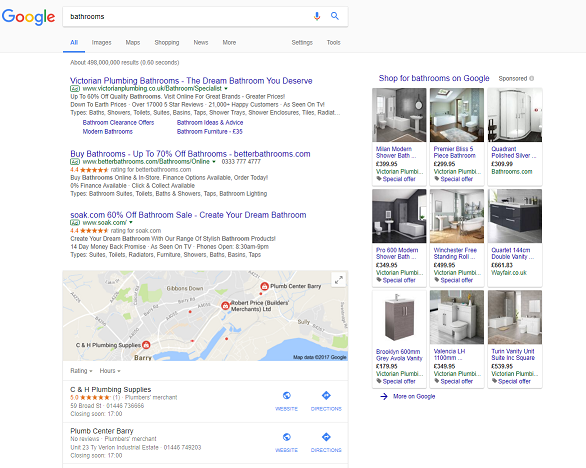A Google search page is displayed with the query "bathroom" entered in the search bar. Below the search bar, options such as "All," "Images," "Map," "Shopping," "News," "More," "Settings," and "Tools" are available. The search results show approximately 498 million results. The first advertisement highlights "Victorian plumbing" with a promise to help create "the dream bathroom you deserve," offering up to 60% off on quality bathroom products. Another promotion mentions significant discounts up to 70% off at "Better Bathroom," encouraging users to "create your dream bathroom." Below the advertisements, there is a map with three location pins identifying places like "G&H Plumbing Supply," "Plum Center," and "Berry." On the right side of the search results, there are images displaying various bathroom sets available for sale. The page appears slightly blurry, making some text difficult to read.